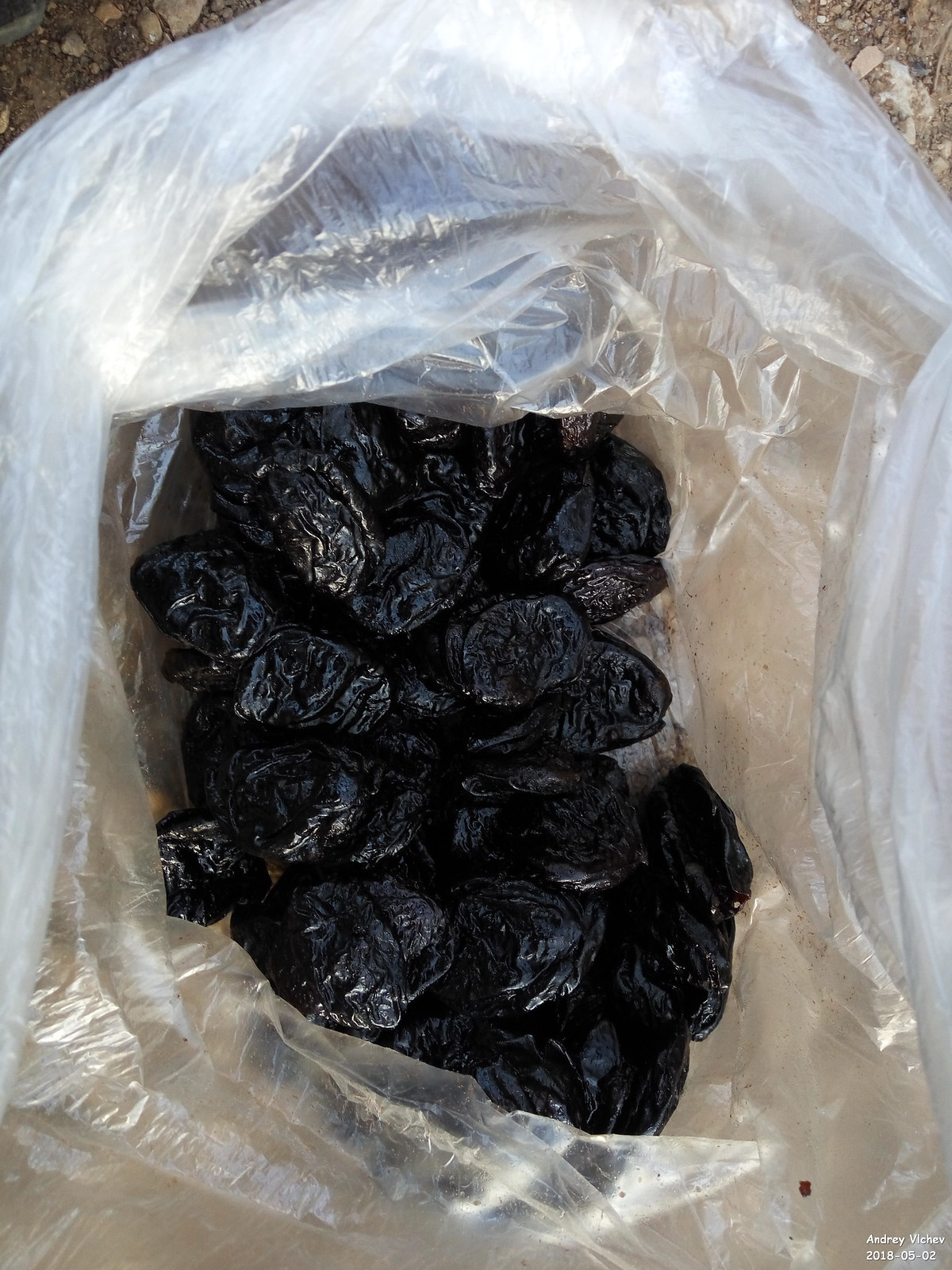This detailed photograph captures a close-up of a clear plastic bag, laid out on a dirt and rock-covered ground. The edges of the image reveal bits of the surrounding earth and stones. Inside the bag, we observe a collection of dried fruits, most likely prunes or dates, numbering around 30 to 35. These fruits are dark, almost black, with a shiny, wrinkly appearance, indicative of either their natural texture or the light reflecting off their surface. The fruits have varied shapes, some rounded and others more irregular. Towards the bottom right corner of the image, the photograph is marked with the text "Andre Vichev 2018-05-02," providing a clue to the image's origin.